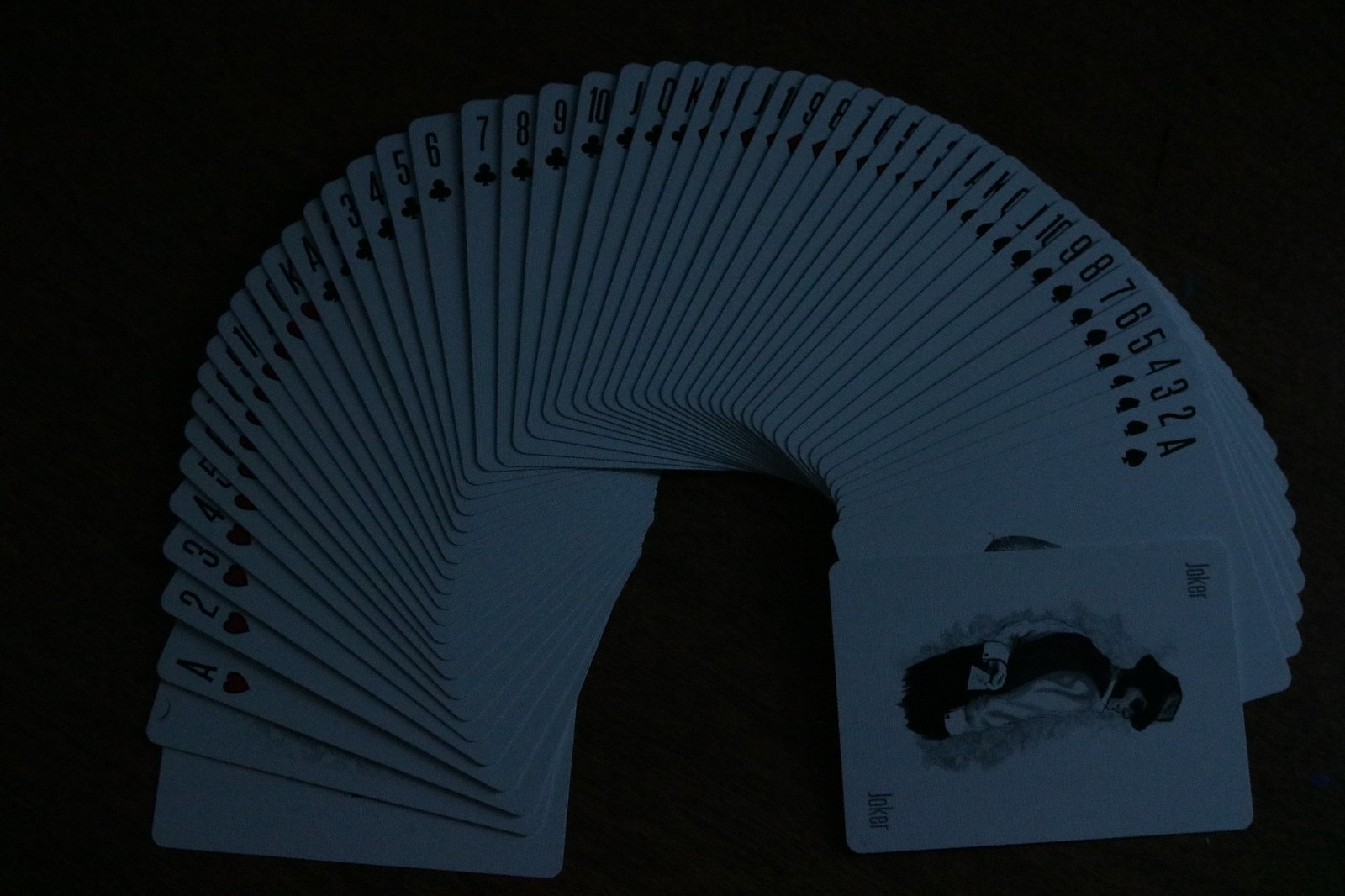The image depicts a deck of playing cards gracefully fanned out in an arc-like arrangement. Each card is stacked atop the previous one, beginning with the bottom card positioned at the lower-left corner of the frame and culminating with the top card at the lower-right corner. 

The foremost card in this elegant display is a Joker, its face turned upward to showcase its white background adorned with dark text reading "JOKER" prominently in both the upper left and lower right corners. Adding a whimsical touch, the card features an illustration of the Joker himself, facing to the right while sporting a distinctive hat.

Immediately behind the Joker card follows the Ace of the deck, succeeded sequentially by the two, three, four, five, six, and so forth. All cards in the series are similarly oriented with their faces visible and pointed upward.

The backdrop of the scene is a solid black color, which enhances the visibility and prominence of the cards. The entire setup is bathed in a dim light with a subtle blue tint, creating a mystical and intriguing atmosphere.